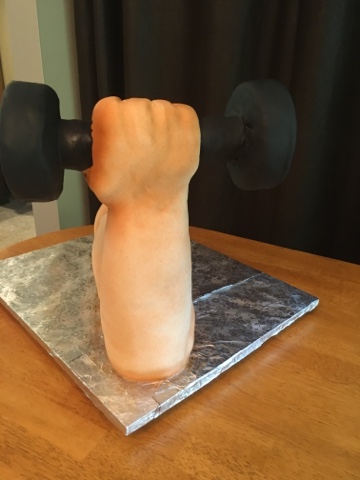The image displays a detailed sculpture of a white-skinned arm in mid-bicep curl, firmly gripping a black dumbbell. The arm is angled upwards, forming a pronounced fist around the dumbbell and terminating at the elbow, which rests on a gray, metallic-looking tile possibly made to resemble foil. The sculpture is placed on a brown wooden table, with a backdrop that includes dark, likely black, curtains and part of a green wall, suggesting a domestic setting. The depiction captures just the arm and dumbbell, with no visible shoulder, torso, or head, presenting a close-up, frontal view of the bicep. This setting creates a focused yet ambiguous form, as the background details and the sculpted, potentially painted nature of the piece blur the lines between reality and art.